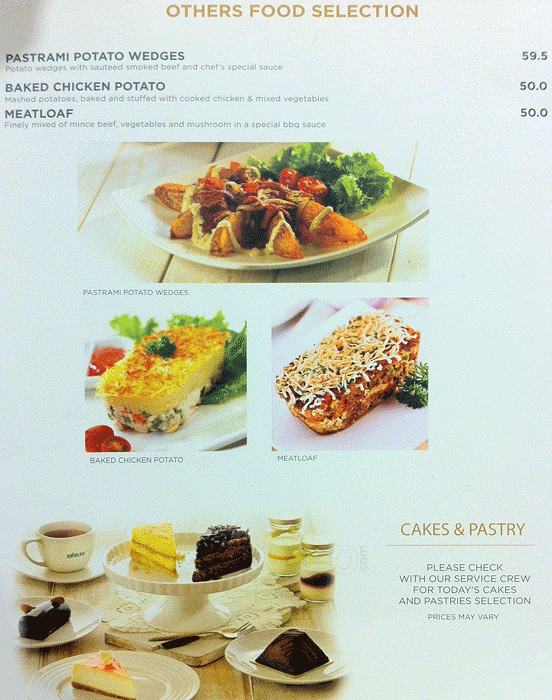This image portrays a detailed food menu with a light blue background. At the top-middle, the title "Others Food Selection" is prominently displayed in orange. The menu lists three main food items: "Pastrami Potato Wedges," described as potato wedges with sautéed smoked beef and the chef's special sauce, priced at 59.5; "Baked Chicken Potato," which includes mashed potatoes baked and stuffed with cooked chicken and mixed vegetables, priced at 50.0; and "Meatloaf," a finely mixed blend of minced beef, vegetables, and mushrooms in a special barbecue sauce, also priced at 50.0. Below these descriptions, there are four food images, showing the listed dishes. To the right side of the last food item, there is a section titled "Cakes and Pastry" with an advisory to check with the service crew for today's selection, noting that prices may vary. The background of the menu is light beige, and the photos depict the dishes in various serving dishes and trays, including coffee cups, cakes, and what appears to be pie, enhancing the visual appeal of the offerings.